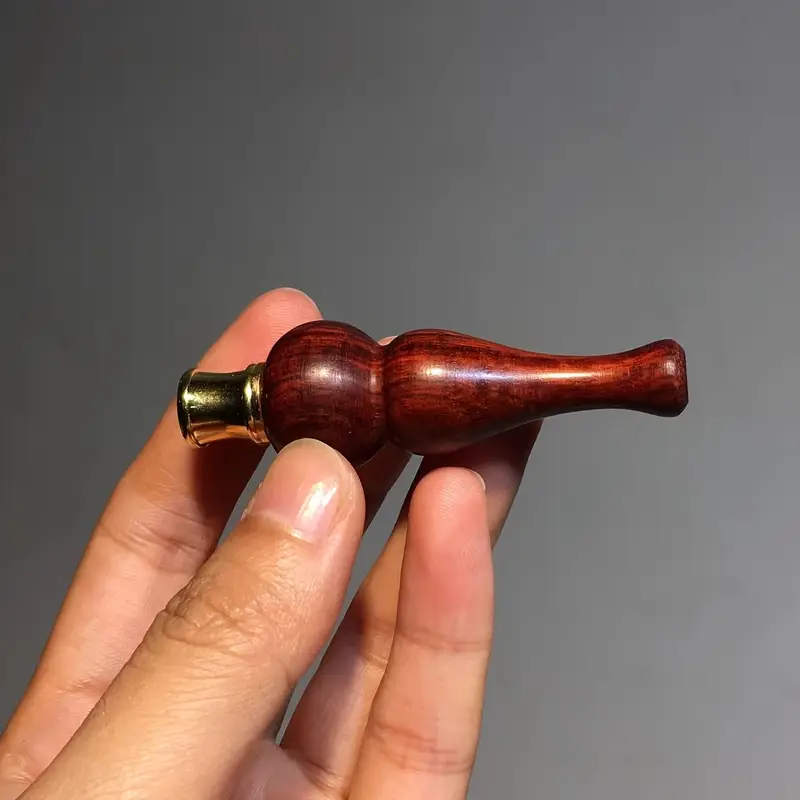In the image, a close-up of a well-manicured hand is seen against a plain gray background. The hand is holding a carved wooden object that has a complex shape. The object, which appears to be made from cherry or rosewood, starts with an oblong, almost interrectangular section that widens into a more circular shape before being cinched and then expanding into a round ball. At the end of this wooden section is a metal tip, likely brass or gold in color, giving it a polished finish. This device, possibly a duck call or similar instrument, seems to be held between the thumb and fingers, with the person's thumb prominently in the foreground.